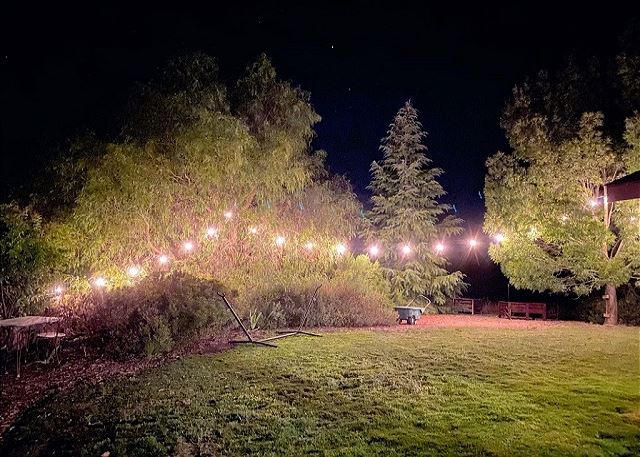The image depicts a vibrant nighttime photograph of an expansive backyard merging into a field, illuminated by a string of globe lights strung in a flowing pattern between trees. The grassy lawn transitions into mulch landscaping, with several species of trees, including evergreens and pines of varying shades from forest green to yellowish-green, creating a rich and textured natural backdrop. In the top section of the photograph, the deep black-blue sky is sprinkled with stars, contrasting sharply with the brightly lit yard below. Notable elements within the scene include a small table with a push-in chair on the left side, a gray wheelbarrow with two large black wheels, a small brown fence with a gate, and a green spreader on wheels slightly off-center to the right. Additionally, there are benches under the trees on the right and a hammock stand without a hammock on the left, enhancing the setting’s cozy, lived-in feel. This detailed composite portrays a harmonious blend of serene natural beauty and thoughtful human touches, captured with photographic realism.